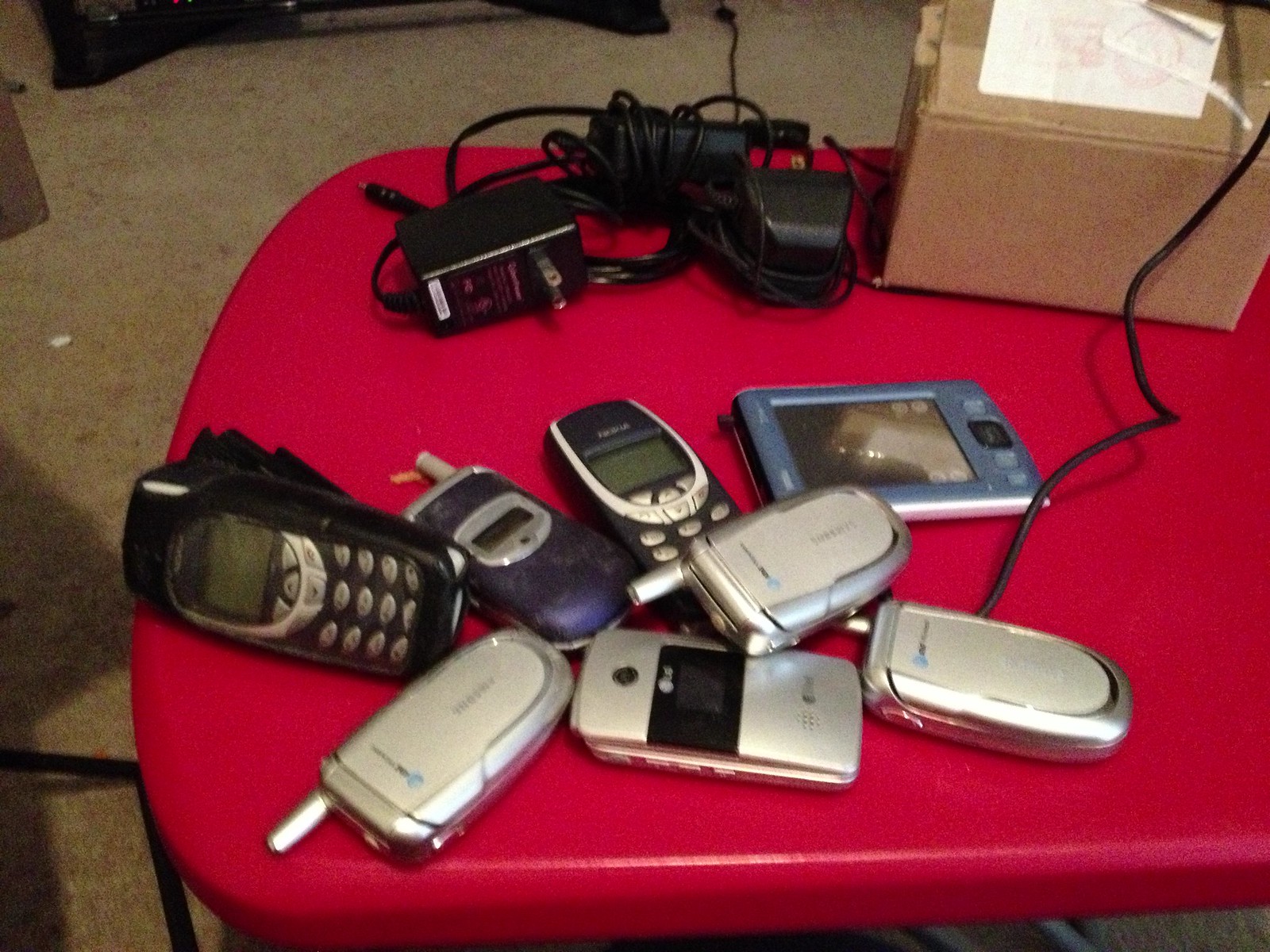The color photograph captures a cluttered indoor scene viewed from above, featuring a dirty wall-to-wall light brown and tan carpet. In the top left corner of the image, partially visible black and brown furniture legs can be seen. Dominating the foreground is a red tabletop with curved corners, possibly part of a chair. Scattered across the table are various old electronic devices, primarily consisting of seven vintage flip phones and one unidentified flat device, which might be an early smartphone, tablet, or handheld gaming device. The flip phones are a mix of silver, black, and dark blue, with many featuring small nub antennas. Accompanying these devices is a small cardboard box with a label, positioned in the upper right corner of the table, and several chunky black power cords and adapters. The photograph possibly captures these items for the purpose of selling or displaying them.